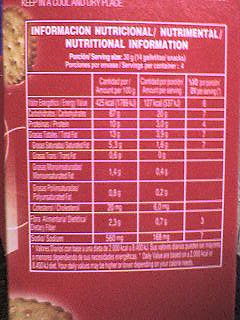This image captures the side panel of a vibrant red box of crackers. On the top left and bottom left corners, there are partial photographs showcasing the crackers themselves. Dominating the center of the image is a detailed nutritional information table, presented in three languages. The top section of the table prominently displays the title "Nutritional Information." Directly below the title, the serving size is indicated in grams, as well as the total number of servings per container. The table is divided into three distinct columns, each providing comprehensive statistics on various nutritional components such as proteins, fats, and other essential nutrients, specifying the amounts present in each serving.